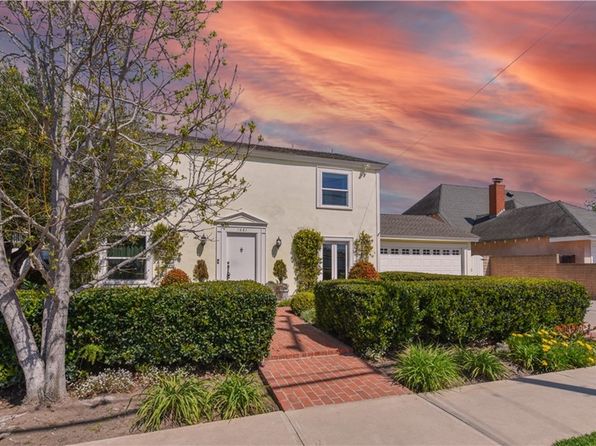The image depicts a standard suburban, two-story home with a pale yellow exterior, situated on a corner lot. The house showcases a white front door with a triangular architectural feature above it, accented by a red brick path leading from the sidewalk to the entrance. The attached garage sits to the right side of the house. Adding to the curb appeal is a hedgerow of neatly trimmed, mature bushes about four feet in height, parallel to the sidewalk and flanking the brick pathway. A large tree in full bloom stands in the front yard, indicating that it is likely spring or summertime. 

The neighboring house to the right is two-story, constructed of red brick with a prominent red chimney. The scene is set around dusk with an orangey cloud cover overhead, featuring pink, purple, and blue streaks reminiscent of stretched cotton candy. The sky's colors accentuate the tranquil, picturesque setting of this suburban neighborhood.